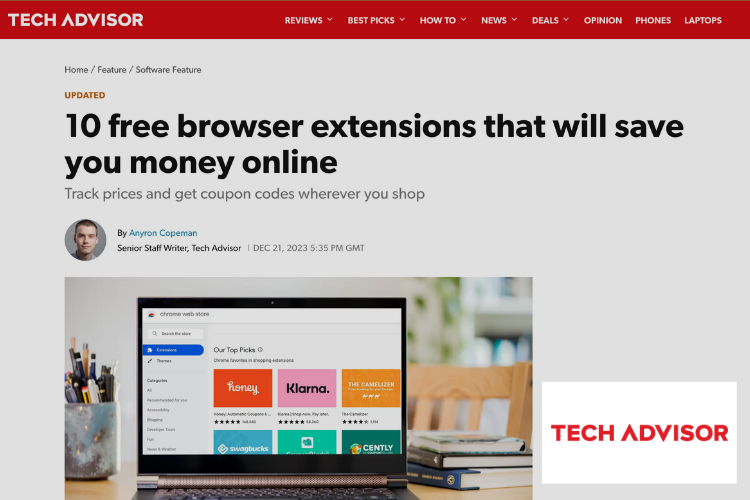This image is a detailed screenshot of a Tech Advisor article from a news website, displayed in a horizontal rectangular frame resembling a computer screen. The top section features a prominent red banner with the "Tech Advisor" logo in white on the left, followed by a menu with drop-down items labeled Reviews, Best Picks, How To, News, Deals, Opinion, Phones, and Laptops. Beneath this, light gray breadcrumbs trace the navigation path: Home > Feature > Software Feature. A category tag above the headline reads "Updated" in brown text.

The main headline, in large black font, announces "10 Free Browser Extensions That Will Save You Money Online," with a subheading that elaborates, "Track Prices and Get Coupon Codes Wherever You Shop." Author information appears below the headline, featuring a small circular avatar beside the byline, "By Anyron Copeman, Senior Staff Writer, Tech Advisor, December 21, 2023, 5:35 PM GMT." The author's name is clickable and highlighted in blue.

Underneath the author information, there's a photograph featuring an open laptop on a desk, displaying the Chrome Web Store with various browser extensions. The desk also holds stacked books and a pencil holder to one side. An advertisement on the right sidebar shows a white rectangle with the red text "Tech Advisor."